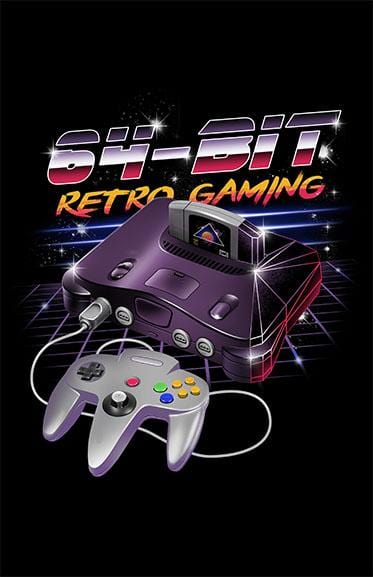The image depicts a computer rendering of a retro gaming console, prominently a Nintendo 64, set against a solid black background. The console, a striking combination of purple and red hues, is centrally positioned and viewed from a slightly elevated angle, revealing both the front and the top. Inserted into the console is a game cartridge, distinguished by its silver-purple color and a central black label. Connected to the console is a classic gray Nintendo 64 controller with three prongs and a matching silver wire.

Above the console, the text "64-bit" is displayed in a mix of red, white, and blue (or sometimes silver and red depending on the rendition) colors. Directly below, the phrase "Retro Gaming" appears in vibrant yellow and pink (alternatively orange) text. Additional design elements include a slight grid pattern and three light blue horizontal lines underneath the "Retro Gaming" text, adding a sleek, modern touch to the nostalgic theme of the poster.